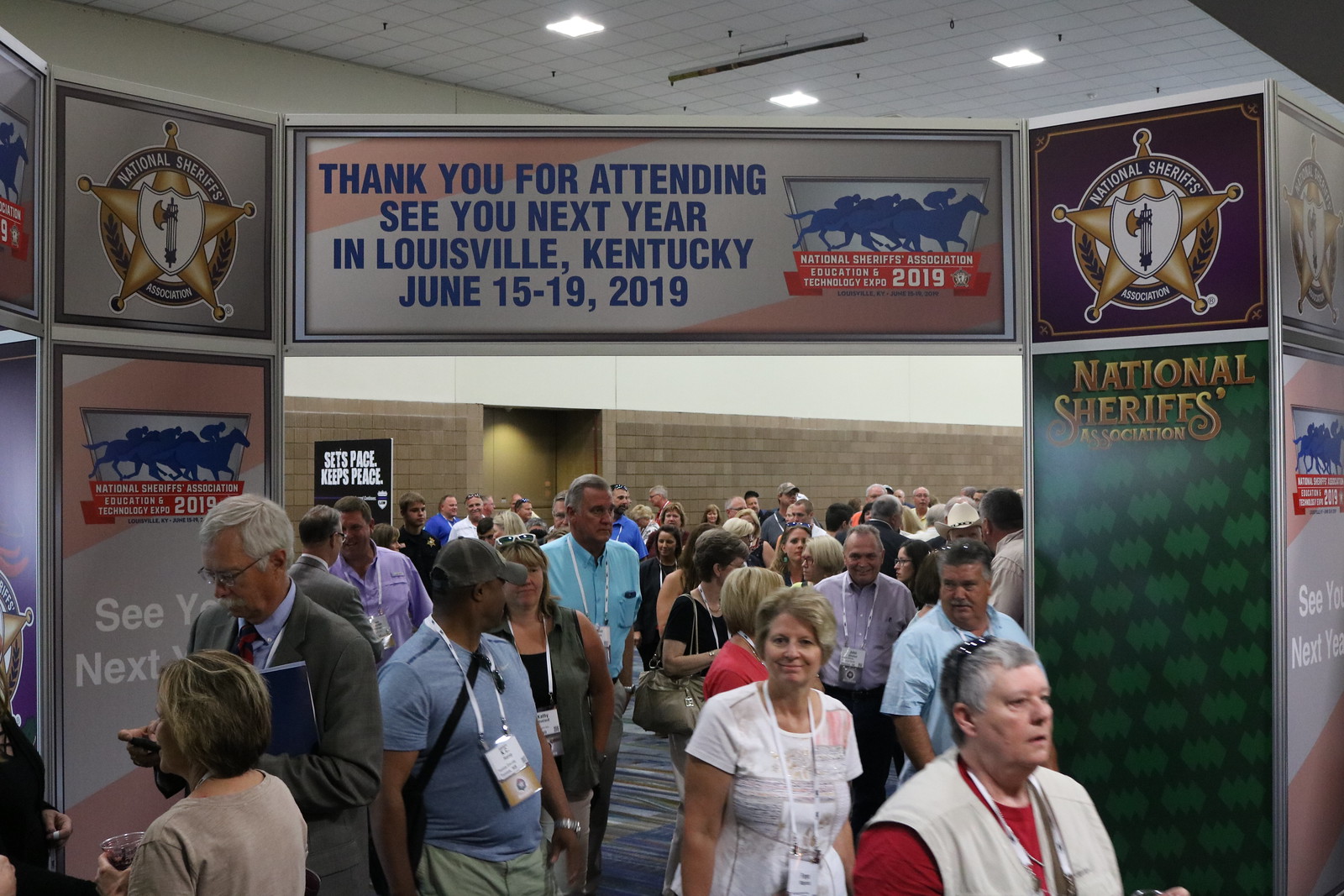The image captures a bustling scene of attendees exiting a large indoor hall at a convention center. The crowd, numbering in the dozens, is comprised of individuals wearing lanyards with identification badges around their necks. Most of them are dressed casually in various colors of short-sleeved shirts, although there is at least one person who is smartly dressed in a gray suit, blue shirt, and red tie. The floor is carpeted, and the people are moving through an archway. A prominent sign above the archway reads, "Thank you for attending. See you next year in Louisville, Kentucky, June 15-19, 2019." Additional text on the sign mentions "National Sheriff's Association Education and Technology 2019," and the organization’s logo, a star, is displayed in the top left and right corners. This detail, combined with a picture of horse racing on the sign, suggests that the event might be linked to both horse racing and the National Sheriff's Association. The vivid array of colors in the attendees' clothing and the signage creates a vibrant atmosphere that indicates the conclusion of a significant event.